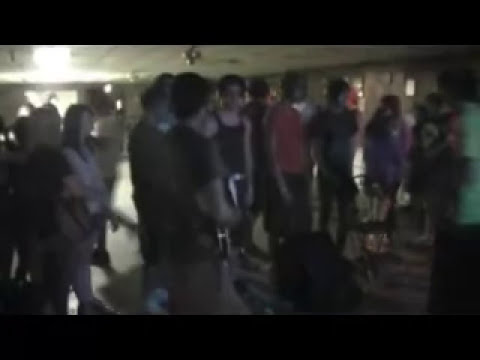This photograph is dark and blurry, capturing an indoor scene with approximately 20 people who appear to be teenagers. The setting seems to have a low, yellowish-beige ceiling, possibly indicating a basement environment. The light source from the upper left corner poorly illuminates the space, adding to the dimness. 

Most of the individuals are dressed in short sleeves or tank tops, suggesting it might be warm in the room. The crowd is largely dressed in black, with 70% of the shirts being that color, while a few others sport distinct hues such as one person with a green shirt and another with a purple shirt. The person in the middle stands out due to a black tank top, and there's someone wearing a red shirt who appears to be pushing a black baby carriage, though it's hard to see clearly due to the blurriness.

The people are mostly facing towards the right side of the image except for the person in the green shirt, who faces them. In front of the group, there is a black square object that might be a speaker, and to the right, there is a wooden chair. Despite the poor quality of the photo, the sense of a crowded, active indoor space is evident.